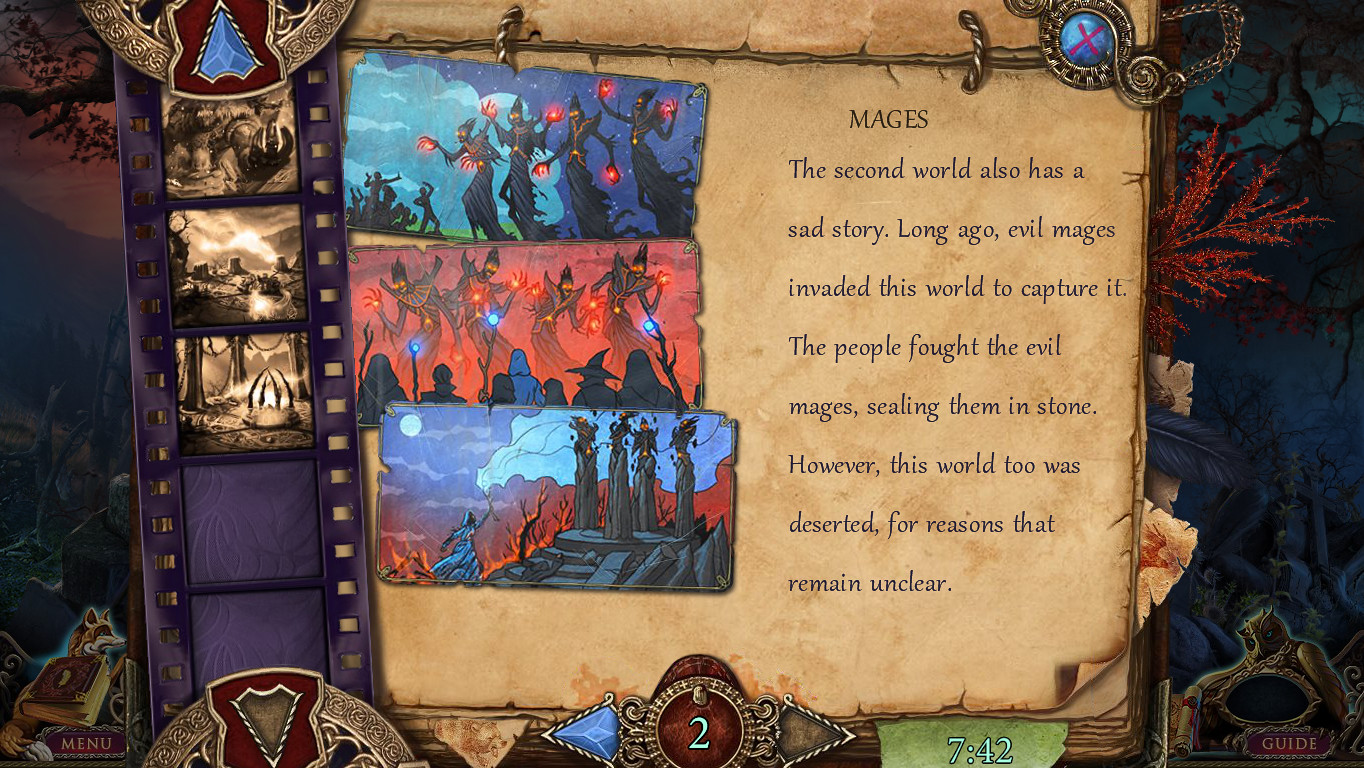The image depicts a fantastical, game-like scene set against a wooded background with tree limbs and leaves. To the left, a purplish-black film strip displaying three indistinct brownish images is partially blank in some areas. On the right, an old, open book tied together with strings contains several colorful illustrations and notes about mages.

At the top section of the page, there are three haunting images of towering figures with red light emanating from their hands and small, frightened people at their feet. Another illustration beneath shows a similar scene, with these ominous figures facing people wearing witch hats and holding staffs emitting blue energy. Further down, a column-like formation consists of four figures atop stairs, with a person running towards them with an outstretched wand. The page is marked with cryptic numbers "2; 742."

On the bottom left, there's a glowing fox with a book labeled "menu" hovering over its body. On the opposite side, an ivory hawk with a mysterious teal glow around its eyes is labeled "guide." The middle of the scene illustrates an elaborate backstory with references to "mages." It recounts a tale of evil mages invading the second world, where people turned them into stone, yet the world remains deserted for unknown reasons. The overall style is cartoonish and imbued with a mystical, old-world fantasy vibe.